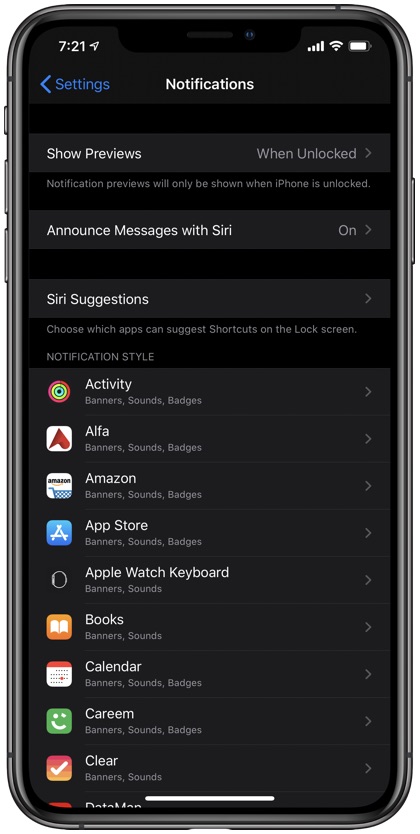A screenshot of a smartphone, which appears to be an iPhone, displays a detailed settings screen. The device has a black bezel with a small button near the upper left side and two larger buttons beneath it, while another larger button is on the right side.

At the top of the screen, the time reads 7:21 in black text, accompanied by a GPS icon. On the right side, icons indicate full cell signal, WiFi connectivity, and a fully charged battery. Below this is a back arrow pointing to the left, alongside the word "Settings" in blue.

The central part of the screen features the word "Notifications" in white. Directly beneath is a gray bar with "Show Previews" written in white on the left and "When Unlocked" on the right. Another gray bar below provides an explanation in gray text: "Notification previews will only be shown when the iPhone is unlocked."

Following this, a gray section on the left reads "Announce Messages with Siri" in white, with the word "On" displayed in gray on the right. Beneath this, another option in gray has "Siri Settings" on the left with an arrow pointing to the right.

The final section reads "Choose which apps can notify you" and lists several applications under "Notification Style," including Activities, Alpha, Amazon, App Store, Apple Watch, Keyboard, Books, Calendar, CARM, and Clear, each with a gray arrow pointing to the right beside it.

This concludes the detailed view of the smartphone settings screen.